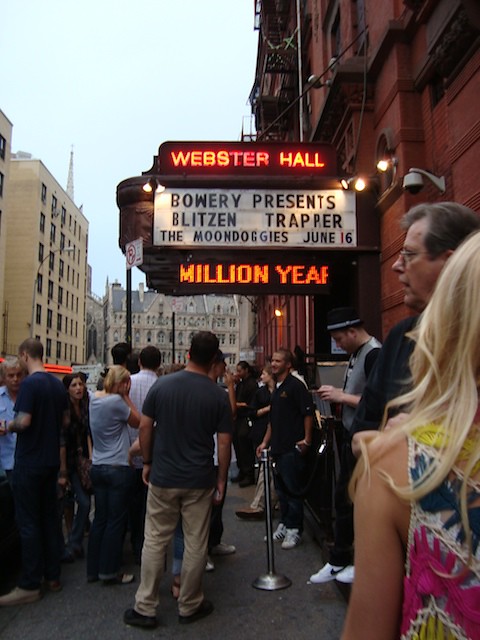The image depicts a vibrant scene on a New York City sidewalk, bustling with people dressed in casual summer attire, standing in line to enter a venue. In the immediate foreground, a blonde-haired woman stands out among the crowd. To the right, the entrance to Webster Hall is highlighted by a prominent red neon sign and a white marquee. The marquee in black letters announces the event: "Bowery Presents Blitzen Trapper the Moondoggies June 16th." Below this, red digital letters display "million year." The venue is housed in a charming, old-fashioned red brick building. In the background, there’s a tall, square, beige building with windows on the left and a more ornate beige building with a peaked roof, numerous windows, and arches in the far distance. The scene captures the lively anticipation of concert-goers on a pleasant summer day.